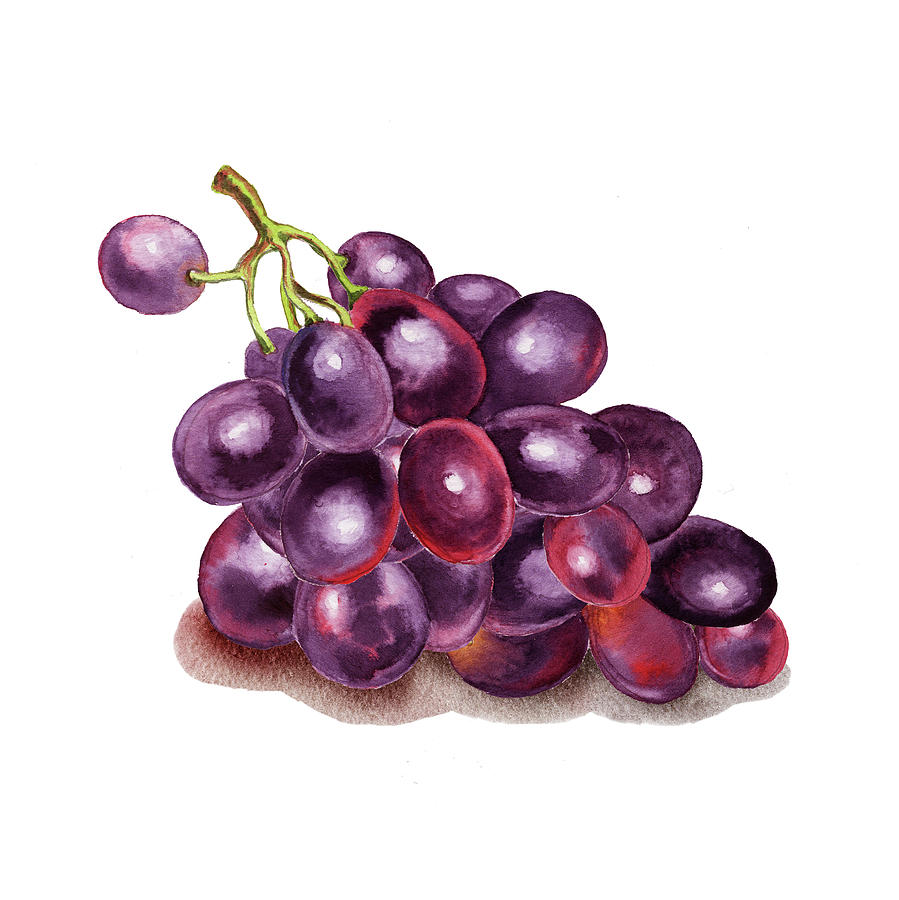This is a watercolor painting of a bunch of purple grapes sitting on a white surface, with no background. The grapes are still attached to a green stem, and a singular grape near the top juts out sideways to the left while the rest of the grapes rest upon each other, creating a densely packed cluster. The grapes exhibit various shades of purple, with some displaying a reddish tint, particularly towards the center and bottom of the bunch. The artist has skillfully painted light reflections on many of the grapes, creating a shiny appearance. The shadows cast by the grapes have a brownish color mixed with hints of red, adding depth and realism to the image. Overall, the meticulous detailing and use of light and shadow give the painting a lifelike quality.